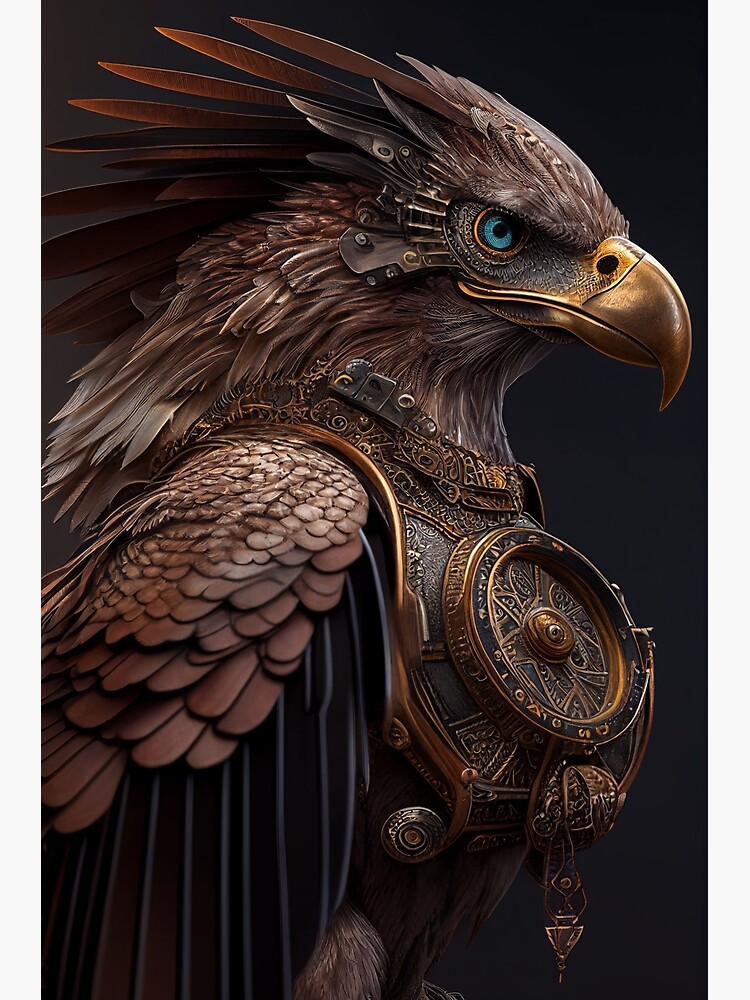This image is a highly detailed, digital rendering of a hawk, possibly an eagle, that appears to be part of a video game or AI-generated artwork. The hawk is facing right, showcasing its prominent light teal-blue eye and its shiny golden-bronze beak, which tapers to a sharp point and features a black line where it splits. The hawk's head is adorned with dark brown feathers, arranged in a way that gives the appearance of a mohawk, while its neck and forehead also display shades of brown. 

Strikingly, the hawk is adorned with a sophisticated, armor-like breastplate made of bronze and black materials. Central to this armor is a decorative, compass-like circle with intricate embellishments. This circle features a black and gold color scheme, with a gold center highlighted by a silver-colored screw and encircled by a gold ring. The armor and the bird's hybrid metallic feathers lend it an impression of a formidable warbird. The intricacy of the design, though impressive, shows some erratic and imprecise lines, typical of AI-rendered illustrations. The entire scene is set against a dark black background, accentuating the detailed textures of the feathers and armor.